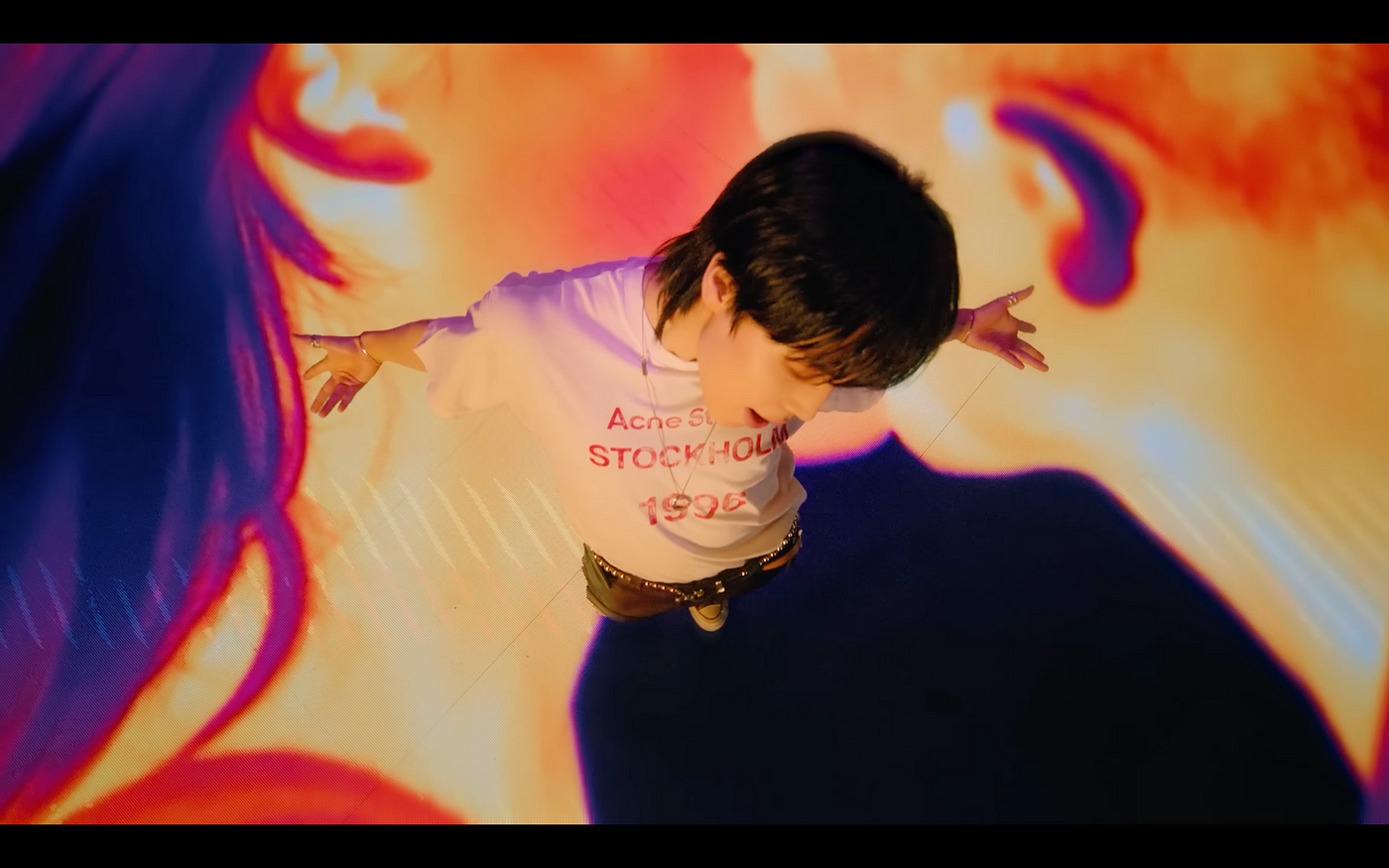This detailed image depicts a young performer, possibly an Asian K-pop artist, captured in what appears to be a scene from a stylized music video. The figure stands alone on a stage or room, with their arms outstretched as if to give a hug, head slightly cocked to one side, seemingly enjoying the moment. The individual is wearing a white t-shirt that features the text "acne Stockholm 1996" and is accessorized with a studded belt, black shorts or jeans, and the visible tip of a white sneaker. The person, who has short black hair, also sports some jewelry on their wrist and fingers. The background is artistically enhanced with superimposed images of two people kissing and vibrant colors like purples, oranges, and yellows, giving it a dynamic and emotional atmosphere. The photo, framed with black bands at the top and bottom, suggests it may be a clip from a video.